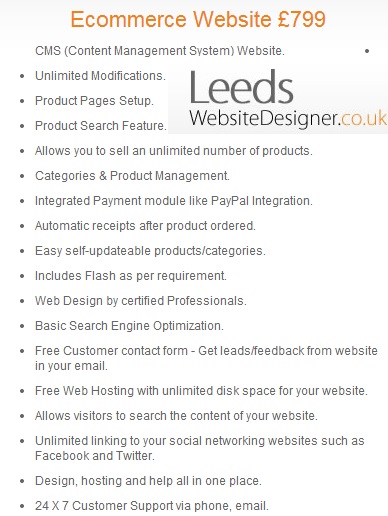This is an advertisement presented on a white background. At the top of the image, "e-commerce website" is prominently displayed in orange text. Below it, the price is indicated as "£799". The ad's core details are listed in smaller black text, starting with "CMS (Content Management System) website". Following this, a comprehensive set of features is outlined through bullet points: 

- Unlimited modifications
- Product page setup
- Product search feature
- Capability to sell an unlimited number of products
- Categories and product management
- Integrated payment module including PayPal integration
- Automatic receipts after product orders
- Easy self-updatable products and categories
- Includes Flash as required
- Web design by certified professionals
- Basic search engine optimization
- Free customer contact form for getting leads and feedback via email
- Free web hosting with unlimited disk space for your website
- Allows visitors to search website content
- Unlimited linking to social networking sites like Facebook and Twitter
- Design, hosting, and support all in one place
- 24/7 customer support available via phone and email

In the upper corner of the advertisement, the service provider's web address "leadswebsitedesigner.co.uk" is displayed. On closer inspection, a gray rectangle adjacent to the top three bullet points highlights this URL, reinforcing the brand identity. The text "leads" appears on one line in dark gray, while "websitedesigner.co.uk" is on the next line, also in dark gray except for "co.uk" which is in a light orange. The background is subtly varied with very light gray for added contrast.